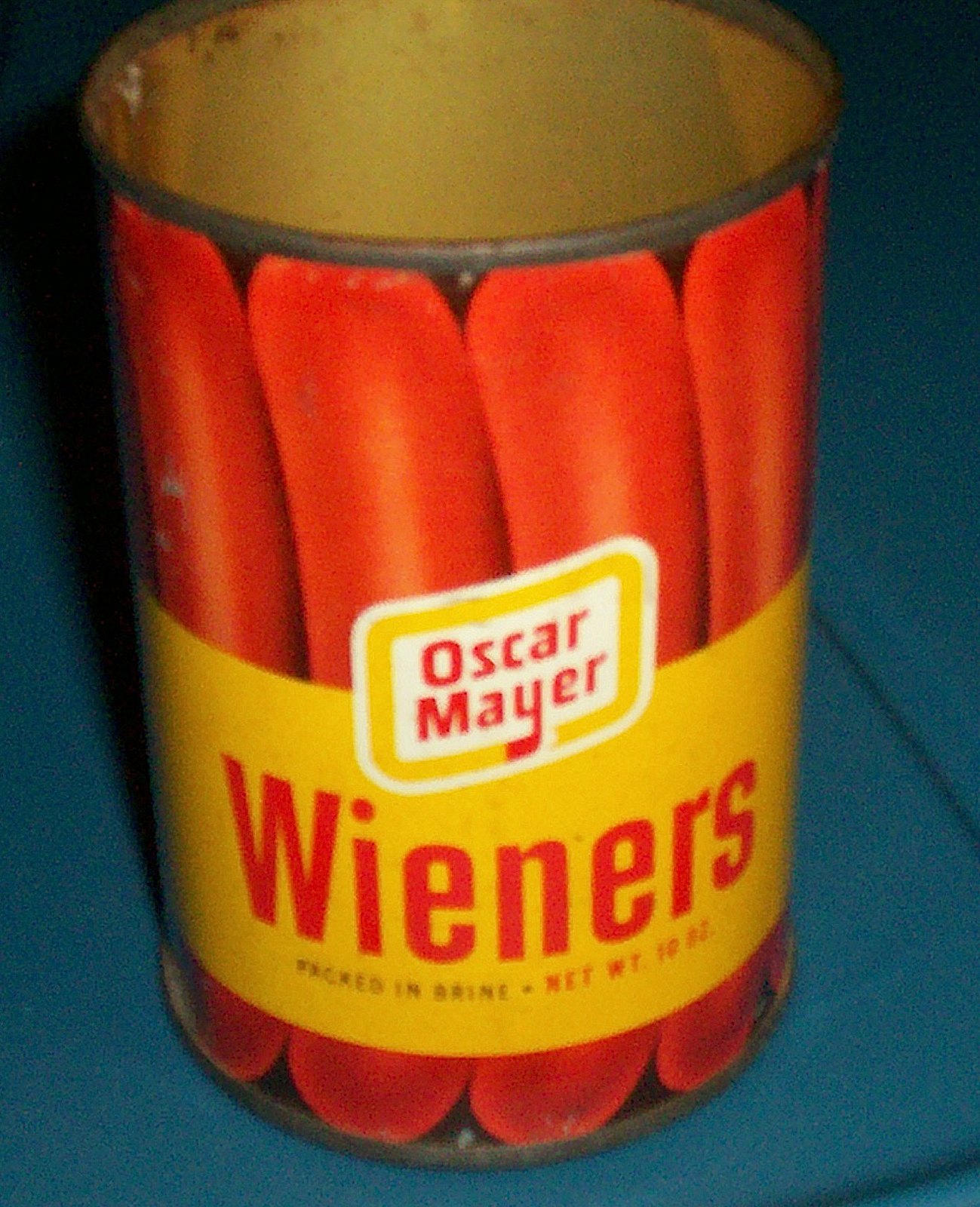The photograph showcases a vintage, empty tin can sitting on a medium-blue surface. The can appears worn with noticeable rust along the top and bottom edges, suggesting significant age. The tin can, which lacks a lid, reveals a tannish-yellow interior. Its label is primarily red and yellow, featuring an image of hot dogs standing upright encircling the can. In the center of the label, a wide yellow band prominently displays the word "Wieners" in orange-red letters. Above this, a diagonal rectangle outlined in white and yellow holds the iconic "Oscar Mayer" logo in red text against a white background. Although the exact net weight is difficult to discern, faint inscriptions hint at “10 ounces”. The old-fashioned design and material of the can, contrasting sharply with modern aluminum cans, further underscore its age, likely dating back to the mid-20th century.